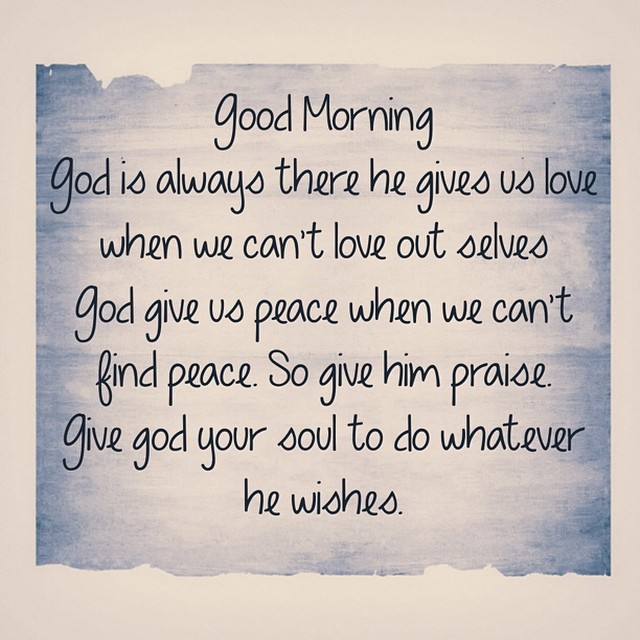This cute and inspirational digital image features a paper-like element situated at the center of a light brown or cream-colored background. The central element has a rectangular shape, although its borders are irregular and torn, giving it a distressed look as if painted with a blue brushstroke that fades to a lighter hue in the center. Over this backdrop, black text in a decorative script font reads:

"Good morning, God is always there. He gives us love when we can't love out ourselves. God gives us peace when we can't find peace. So give Him praise. Give God your soul to do whatever He wishes."

Despite a small spelling error in the word "out" instead of "ourselves," the message remains a heartfelt reminder of divine presence and love, encouraging readers to entrust their souls to God's care.